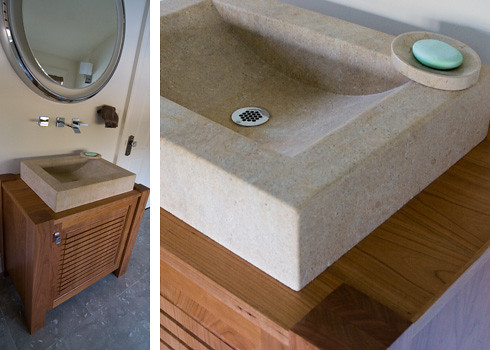This photograph consists of two images displayed side-by-side. 

The image on the left showcases a stylish bathroom vanity area. Dominating this scene is a rectangular sink setup against an off-white wall. Above the sink, an oval-shaped mirror with a sleek silver border is mounted. The mirror reflects a neat rectangular light fixture with a silver body on a white base. Below the mirror, a modern silver faucet with two matching handles stands out. To the right of the faucet, a brown towel hangs, adding a touch of warmth to the setting. The square-shaped sink top, crafted from off-white stone, sits elegantly atop a brown cabinet door featuring horizontal slats.

The image on the right offers a close-up side view of the same sink. Here, the square sink's elegant design is clearly visible, with a silver drain positioned at its center. Positioned in the upper right corner of the sink, there's a matching off-white soap dish holding a green, oval-shaped bar of soap. A glimpse of the wooden furniture supporting the sink adds a cohesive element to the design.